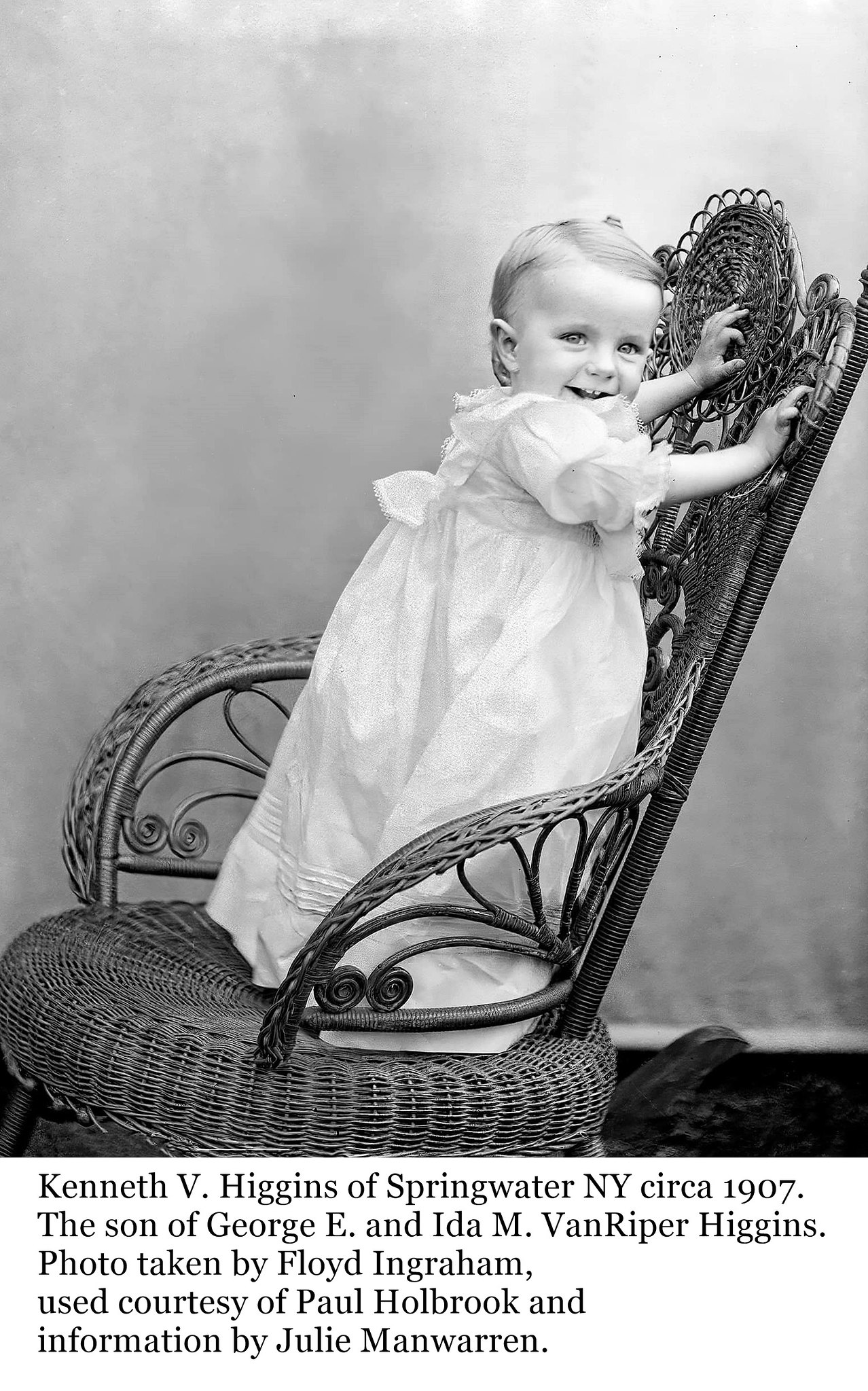This is an old black and white photograph of a smiling toddler named Kenneth V. Higgins of Springwater, New York, taken circa 1907. The photograph depicts Kenneth standing up in an antique wicker armchair, which features a round seat and ornately decorated backing and armrests. The child, dressed in a white ruffled gown with puffy sleeves that reach the elbows, has their hands resting on the back of the chair for balance. The background is a blotchy, grayish-white pattern, typical of early photographic studios. Below the image, there is a white strip containing black text that provides details: "Kenneth V. Higgins of Springwater, New York, circa 1907. The son of George E. and Ida M. Van Riper Higgins. Photo taken by Floyd Ingraham, used courtesy of Paul Holbrook, and information by Julie Manwarren."